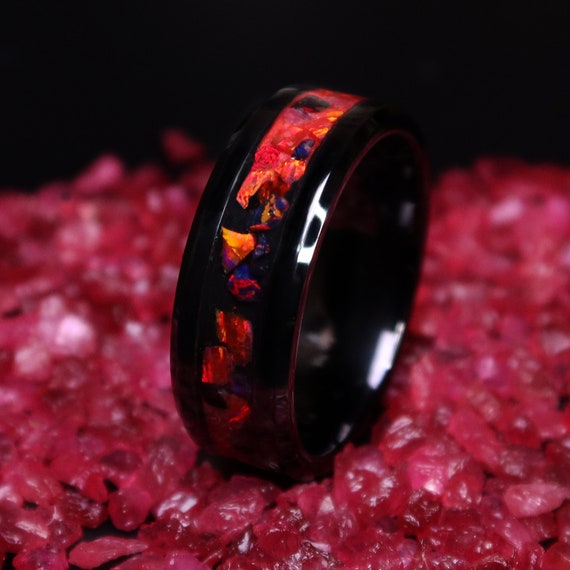The image features a striking man's wedding ring crafted from a shiny black metal, possibly akin to blackened onyx or stainless steel. The design is accentuated by a central band adorned with an intricate array of small, flat crystals in a spectrum of dazzling colors including vibrant reds, purples, oranges, blues, and yellows. This multicolored band bears a visual resemblance to molten lava or crushed crystals, contributing to the ring's unique and artistic appearance. The ring itself is elegantly placed atop a pile of pink, glass-like crystals, adding to the overall allure of the photograph. The background remains a stark, unfocused black, which contrasts sharply with the vibrant colors of the ring and the pink crystals, enhancing the ring's visual prominence and sophisticated charm.